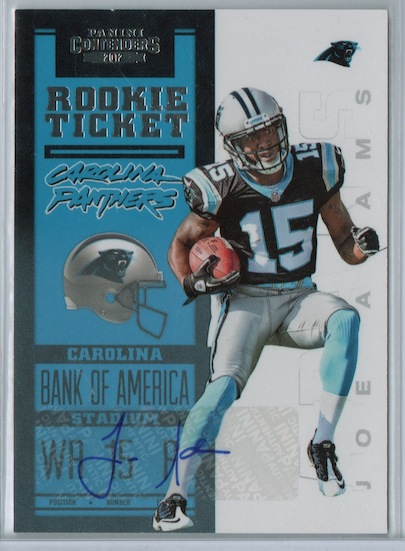This is a detailed football trading card encased in a protective, clear plastic sleeve. The card features a stylized photo of a football player in full Carolina Panthers uniform, holding a football in his right hand, with the jersey number 15 prominently displayed. The left half of the card has a blue background, while the right half is white. At the top left, the card reads "Panini Contenders," though it is somewhat hard to make out, followed by "Rookie Ticket" in silver, uppercase letters. Below this, on a blue banner, is the text "Carolina Panthers" along with the Panther's helmet logo. Further down, the card mentions "Carolina" and "Bank of America Stadium" on a gray background. On the right side of the card, partially obscured by the player's arm, is the name "Joe Adams," with the visible letters being "A" followed by "A-M-S." Additionally, the top right corner of the card features a small image of the Carolina Panthers' logo. The card also includes a signature written in blue sharpie.